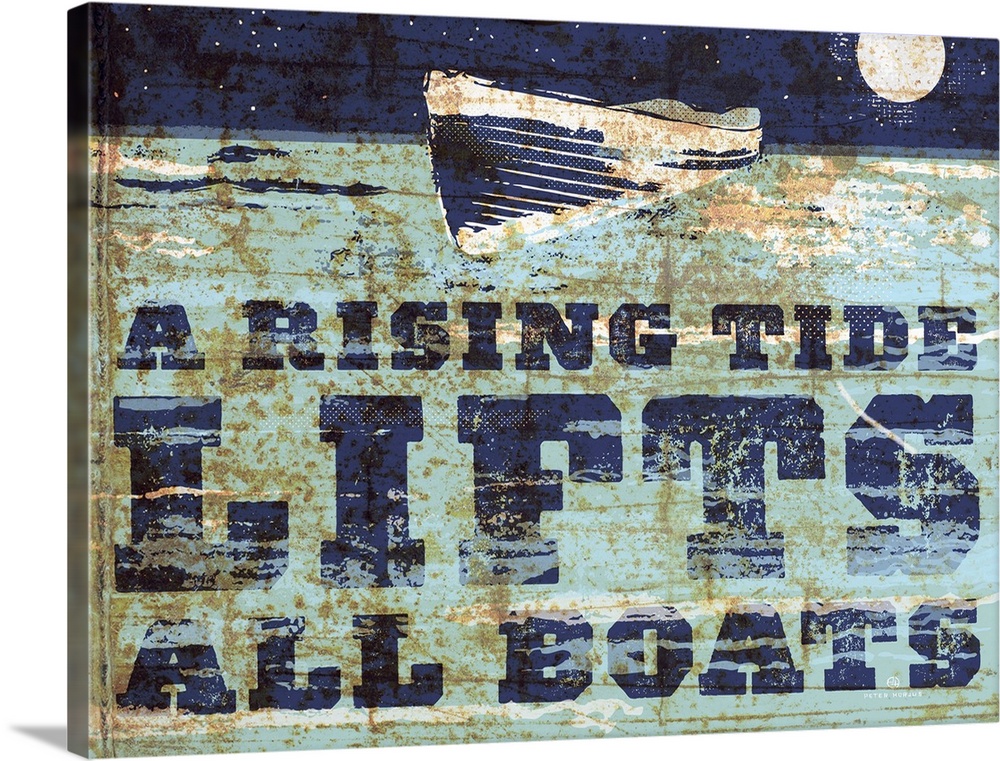The image depicts a rectangular sign, slightly tilted to the right, displaying a weathered, rusted look, giving it an aged appearance. The background features a light blue sea, with darker blue towards the back left, and a dark blue top portion that includes a depiction of a moon in the upper right-hand corner. A detailed boat with blue stripes and a white design also appears on the sign, looking somewhat crusty and worn down, emphasizing the vintage feel. The sign bears the text "A rising tide lifts all boats" in bold, navy blue lettering. The entire composition, possibly made to resemble damaged wood or stone, includes elements that make it look deliberately distressed to suggest it has survived many decades.